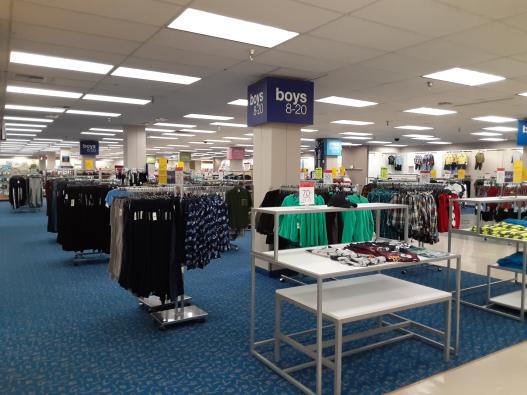This image captures the interior of a retail store from the front entrance, providing a comprehensive view into its layout and atmosphere. In the foreground, there are two multi-level white Formica display tables; the higher table is adorned with neatly laid-out clothing items. Just behind these tables, various racks are filled with women's apparel, featuring an assortment of skirts and tops. The flooring beneath shifts between a blue patterned carpet and white linoleum, creating a visually appealing contrast.

A prominent pillar stands behind the clothing racks, drawing attention with a blue sign that reads "Boys 8 to 20" affixed near the ceiling. This indicates a section of the store dedicated to boys' clothing. Farther into the store, more racks of clothing extend towards the back, demonstrating the store's extensive inventory. Above, bright fluorescent lights housed in ceiling panels provide ample illumination, creating a vibrant and welcoming shopping environment.